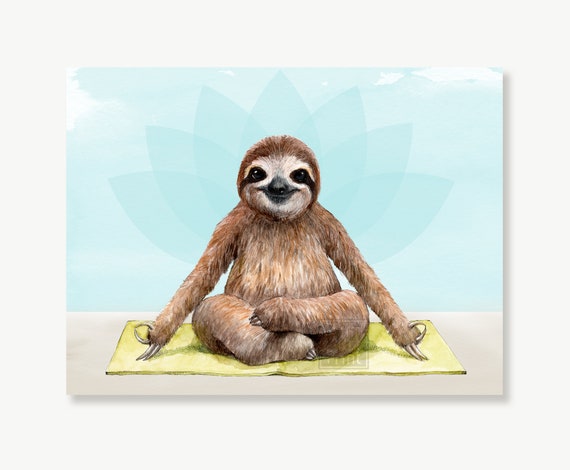This is a vibrant, hand-drawn artwork showcasing a smiling sloth in a meditative yoga pose. The sloth, with its natural brown and white fur, possesses a white face marked by distinctive black, panda-like eyes. It sits cross-legged on a yellow-green yoga mat, hands resting on its knees with thumb and forefinger touching in a traditional meditation gesture. The background features a serene, light blue sky with soft white clouds, painted in a watercolor style. Behind the sloth, an abstract, translucent floral pattern—reminiscent of flower petals—adds an ethereal touch, subtly enhancing the composition. Overall, the piece exudes a calm, pleasing aesthetic, making it an ideal addition to a tranquil space.